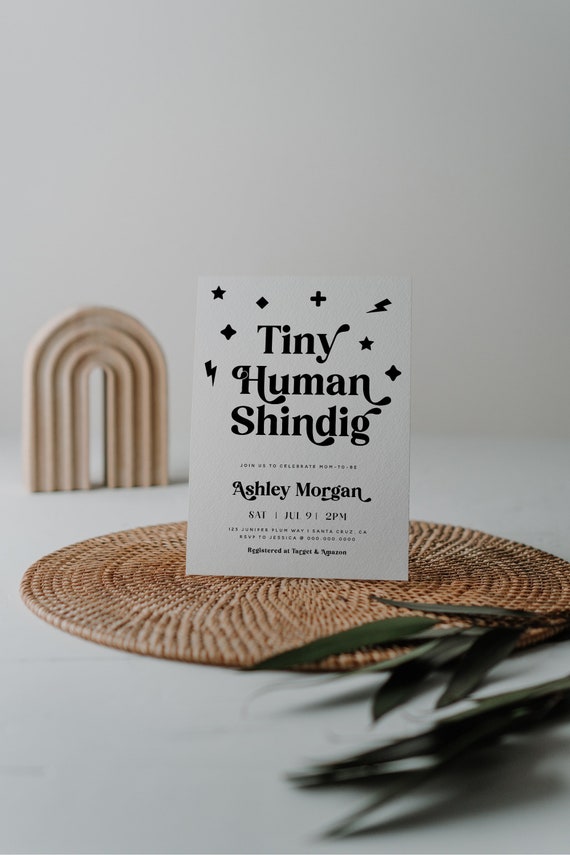In this color photograph, the focal point is a white invitation card placed on a light brown, woven, circular placemat situated in the center of a white table. The card, predominantly white with black text and symbol designs including a lightning bolt, a plus sign, a diamond, and a star, announces a baby shower titled "Tiny Human Shindig" for mom-to-be Ashley Morgan, to be held on Saturday, July 9th at 2 p.m. Below the date, there's additional text which provides further event details and notes registration at Target and Amazon. Surrounding the placemat, two slightly out-of-focus leafy plant stems can be seen at the lower side of the image, casting shadows on the table. In the background, the top part of a ripple-patterned chair is visible, along with a beige, oval, rainbow-shaped standing artwork. Both the chair and the artwork appear slightly out of focus.